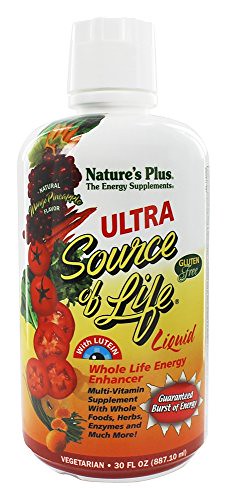A detailed caption for the image:

"Presenting Nature Plus, the premium energy supplement meticulously crafted to boost your vitality. This sleek, white, round bottle is adorned with vibrant, eye-catching designs. Dominating the front label is the bold text 'Nature Plus, The Energy Supplement, Ultra Source of Life Liquid'. Highlighting its potency, the caption 'Whole Life Energy Enhancer' is prominently displayed in red. Beneath, in black, the benefits are elaborated: 'Multivitamin Supplement with Whole Foods, Herbs, Enzymes, and Much More'. 

On the right side of the label, a dynamic sunburst graphic captures attention, with a red core and white text declaring a 'Guaranteed Burst of Energy'. The left side is graced with images of assorted vegetables, including ripe tomatoes, fresh greens like spinach, and juicy grapes, underscoring the product's natural ingredients. 

At the bottom of the bottle, in clean white text, it indicates 'Vegetarian' and specifies the volume as '30 fluid ounces (887.10 milliliters)'. The overall color scheme features an energizing palette of reds, oranges, yellows, and whites, reflecting the supplement's vibrant promise. This product image, set against a plain background, is perfect for an online store, clearly detailing what makes this liquid energy supplement a standout choice."